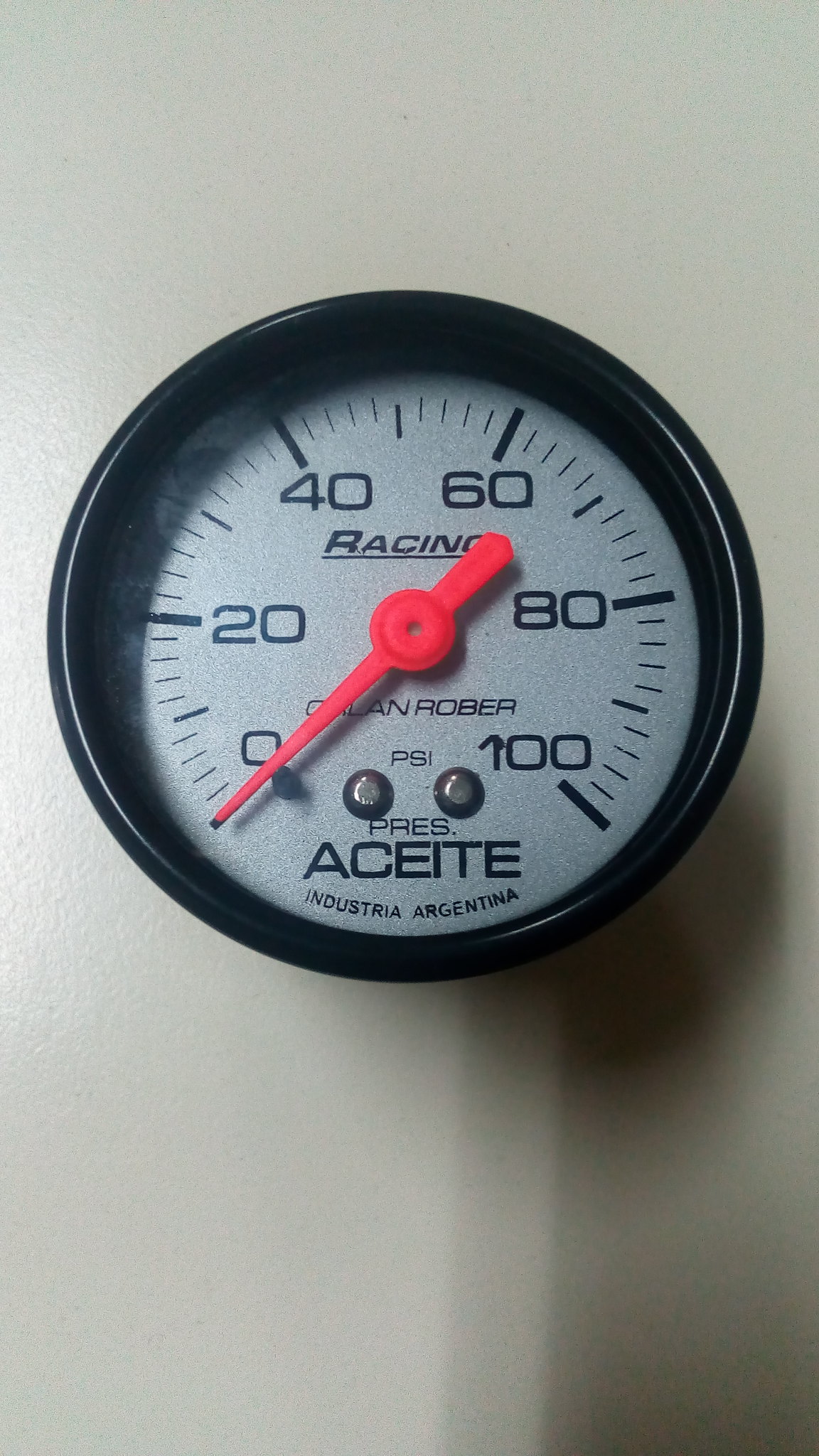A photograph depicting a round pressure gauge with a white background and black markings. The gauge features the word "ACEITE" (Spanish for "oil") prominently displayed, while the top part of the display partially shows the letters "R-A-G-I-N," with the rest obscured. Large numerical indicators read 0, 20, 40, 60, 80, and 100, interspersed with smaller tick marks indicating every two units. The units are labeled in pounds per square inch (PSI). A red pointer indicates the current pressure measurement. The device is mounted with two visible silver screws near the PSI label. The background of the image is plain and indistinct, offering no additional context. The gauge's color scheme is primarily black and white, with a striking red needle for easy reading. This instrument is likely used for measuring oil pressure or a similar application, given the term "ACEITE."